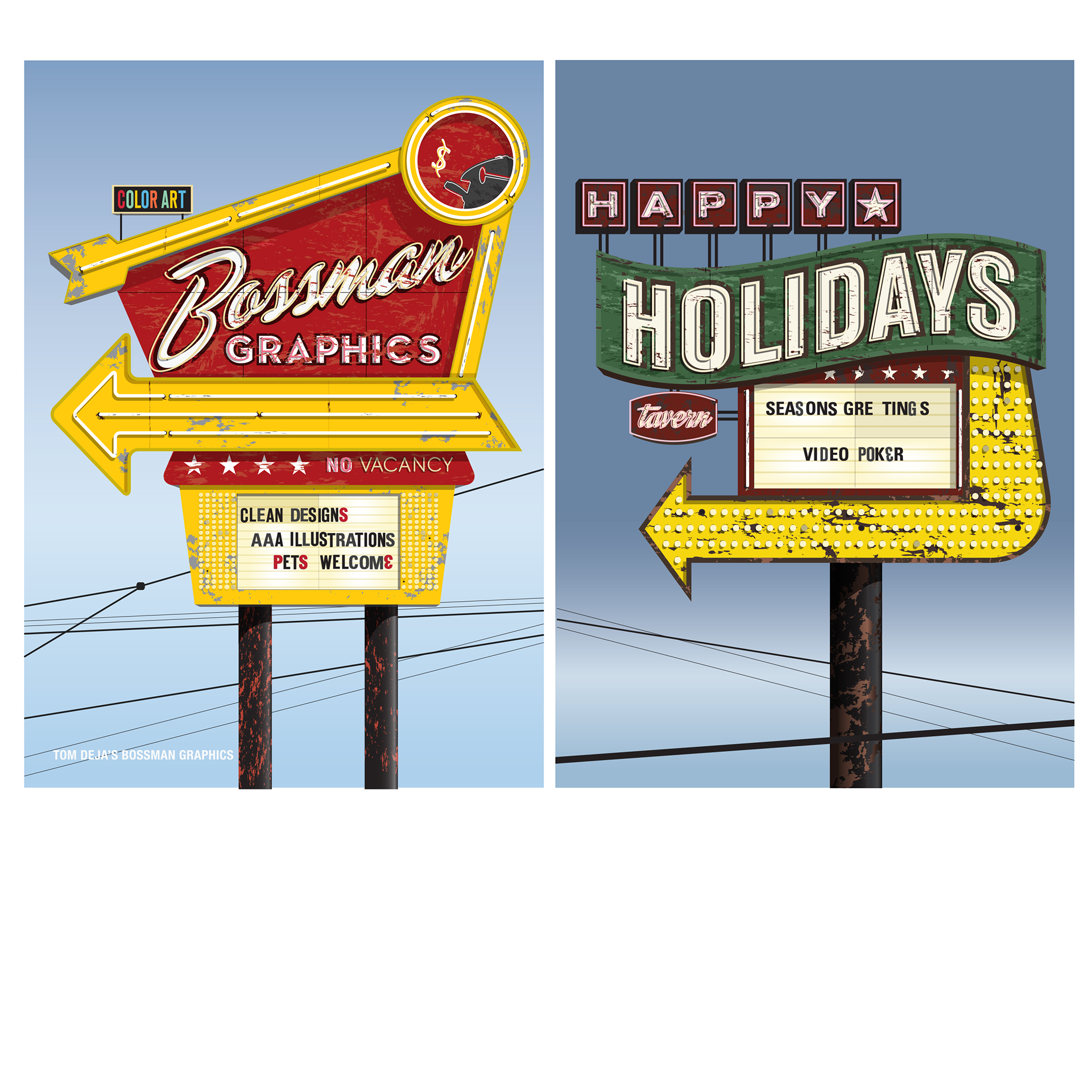This image features two adjacent outdoor scenes, each showcasing different signs mounted on poles with electrical wires and blue sky in the background. The sign on the left, supported by two metal poles, prominently reads "Bossman Graphics" at the top, followed by "No Vacancy," "Clean Designs," "AAA Illustrations," and "Pets Welcome." Additionally, it includes "Color Art" with a depiction of a fish featuring a money sign within a circle, and at the very bottom, the label "Tom Deja's Bossman Graphics." The sign on the right, held up by a single black metal pole, bears the messages "Happy Holidays" in red squares with a white star, "Seasons Greetings," "Video Poker," and "Tavern" with a large illuminated yellow arrow pointing to the left. This comprehensive depiction captures the detailed artistry of Tom Deja's custom signs and designs.